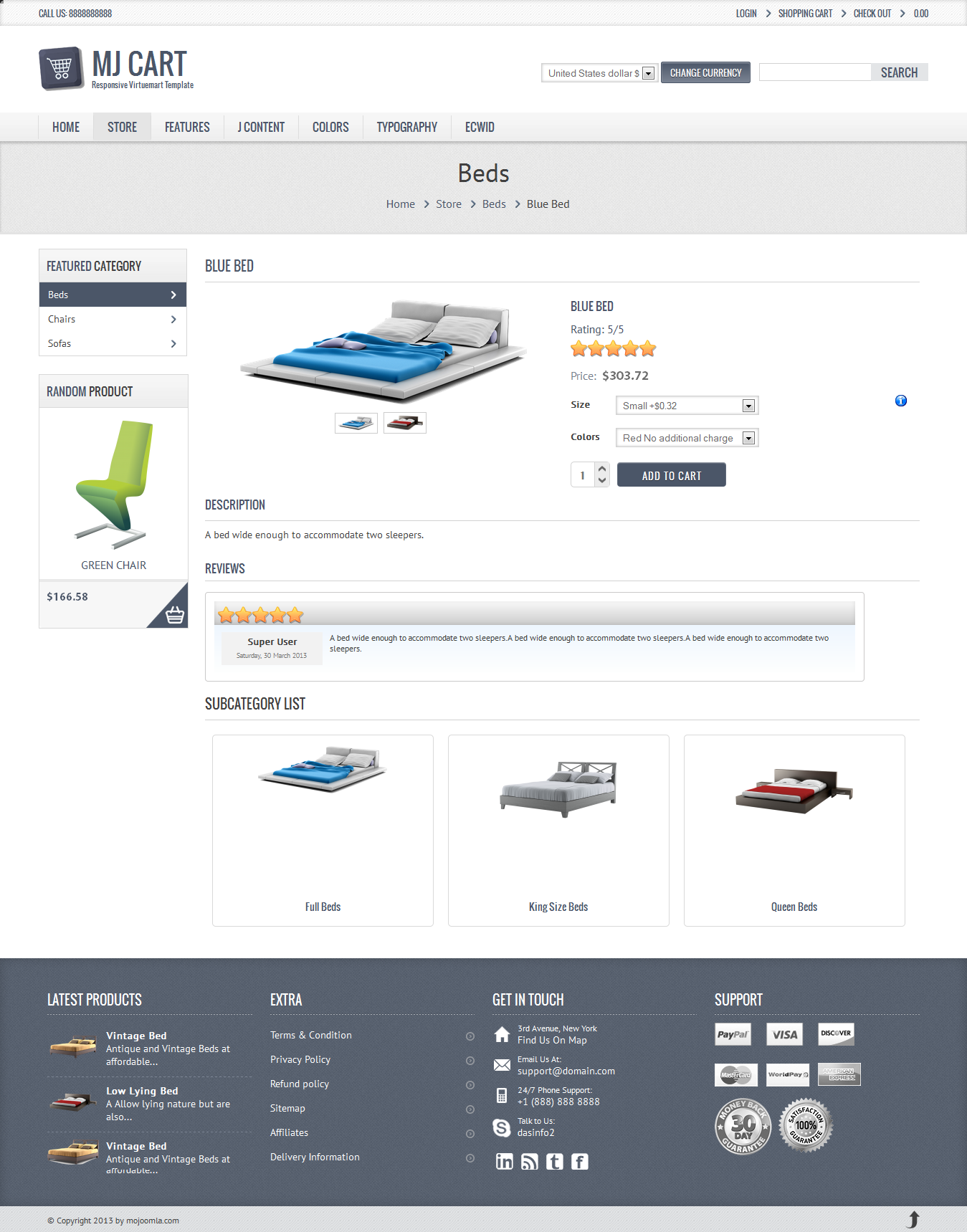Screenshot of the MJCART Responsive VirtuMart Template Generator for a Retail Site

This screenshot showcases the MJCART Responsive VirtuMart Template, a customizable template generator intended for online retail sites. The template simulates a live store setup, although it remains incomplete, as evidenced by placeholder information such as the phone number listed as "888-888-8888" and the email displayed as "support@domain.com."

The primary focus of the site appears to be furniture, with a notable emphasis on beds. The main featured item is a small blue bed, highlighted with a 5 out of 5-star rating and priced at $303. The description notes that the bed is spacious enough to accommodate two sleepers. 

Below the primary product, a subcategory list categorizes additional bed options, such as full beds, king size beds, and queen beds. To the left, in a smaller subcategory section named "Random Product," a green chair is featured, priced at $166.58. 

It is apparent that the products depicted are AI-generated placeholders, serving to illustrate the template's functionality rather than actual items available for purchase.